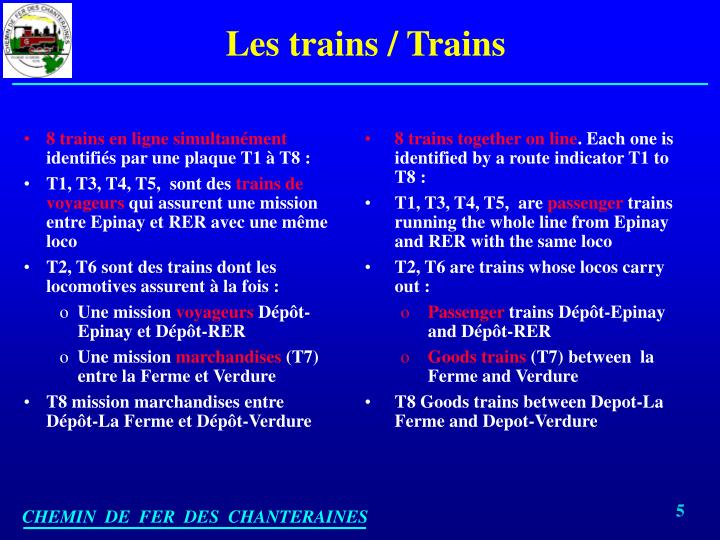The image is a presentation slide from a pamphlet or instructional material on trains, featuring text in both French and English. The slide's background transitions from a lighter blue at the top to a darker blue at the bottom and has a vibrant appearance overall. In the upper left-hand corner, there's an emblem with a red steam train inside a white circle, accompanied by a teal-blue underline beneath the title "Les Trains / Trains," where "Les Trains" appears in yellow font.

The slide content is organized into two columns, with French text on the left and English text on the right. Each language section includes four bullet points, highlighted with red text, detailing information about train routes and their respective functions:

1. **Eight trains together on the line**: Each train is identified by a route indicator, T1 to T8.
2. **Passenger Trains (T1, T3, T4, T5)**: These trains run the entire line from Éponay to RER with the same locomotive (loco).
3. **Passenger Depot Trains (T2, T6)**: These trains' locomotives handle routes from depot Éponay to depot RER.
4. **Goods Trains**: T7 operates between La Ferme and Verdoux, while T8 runs between depot La Ferme and depot Verdoux.

At the bottom of the slide, additional text in blue, possibly a footer, reads "Chemin de fer développement," indicating it might be associated with railway development.